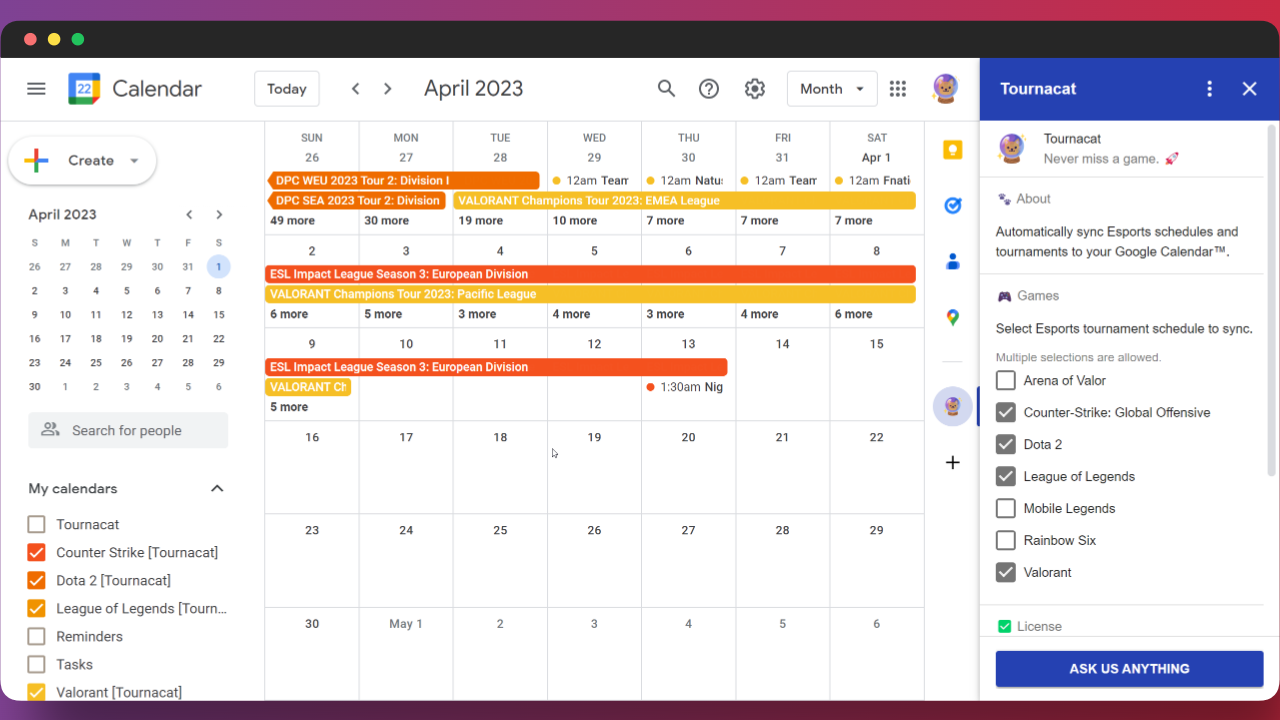This image is a detailed screenshot of a Google Calendar page in landscape mode. 

At the top of the screenshot, stretching from the upper left to upper right, there is a gradient banner starting in purple and transitioning to red. Below this banner, there's a black stripe that features a cluster of three dots in pink, yellow, and green at the center-left. 

Directly beneath the black stripe is a white stripe which contains several navigational elements. From left to right, these elements include: the label "Google Calendar," a "Today" button, a date display showing "April 2023," a search icon, a help icon, a settings icon, a month drop-down menu, and an avatar icon portraying a cat inside a glass bowl.

On the left-hand side of the screen, there is a vertical sidebar that features a mini calendar for the month, alongside a "Create" button for new events and a search bar for finding people. The bottom left section of this sidebar lists various calendars, including "Turnicat," "Counter-Strike," "Dota 2," "League of Legends," "Reminders," "Tax," and "Valorant." Among these, "Counter-Strike" is checked off in red, while "Dota 2," "League of Legends," and "Valorant" are checked off in orange. The other calendars have empty checkboxes.

Moving to the central part of the calendar view, specific events are visible spanning various dates. For instance, from March 26 to 28, there are events indicated by orange lines. From March 28 through April 1, there are events marked with yellow lines. The next row indicates more events, such as the "ESL Impact League Season European Division" in orange and the "Valorant Champions Tour" in yellow.

On the right column, there is a feature titled "Turnicat," which highlights the capability of automatically syncing esports schedules and tournaments to Google Calendar. At the very bottom right corner, there's a prominent blue button labeled "Ask us anything."

This image offers a comprehensive overview of a user's esports schedules, integrated within their Google Calendar interface.